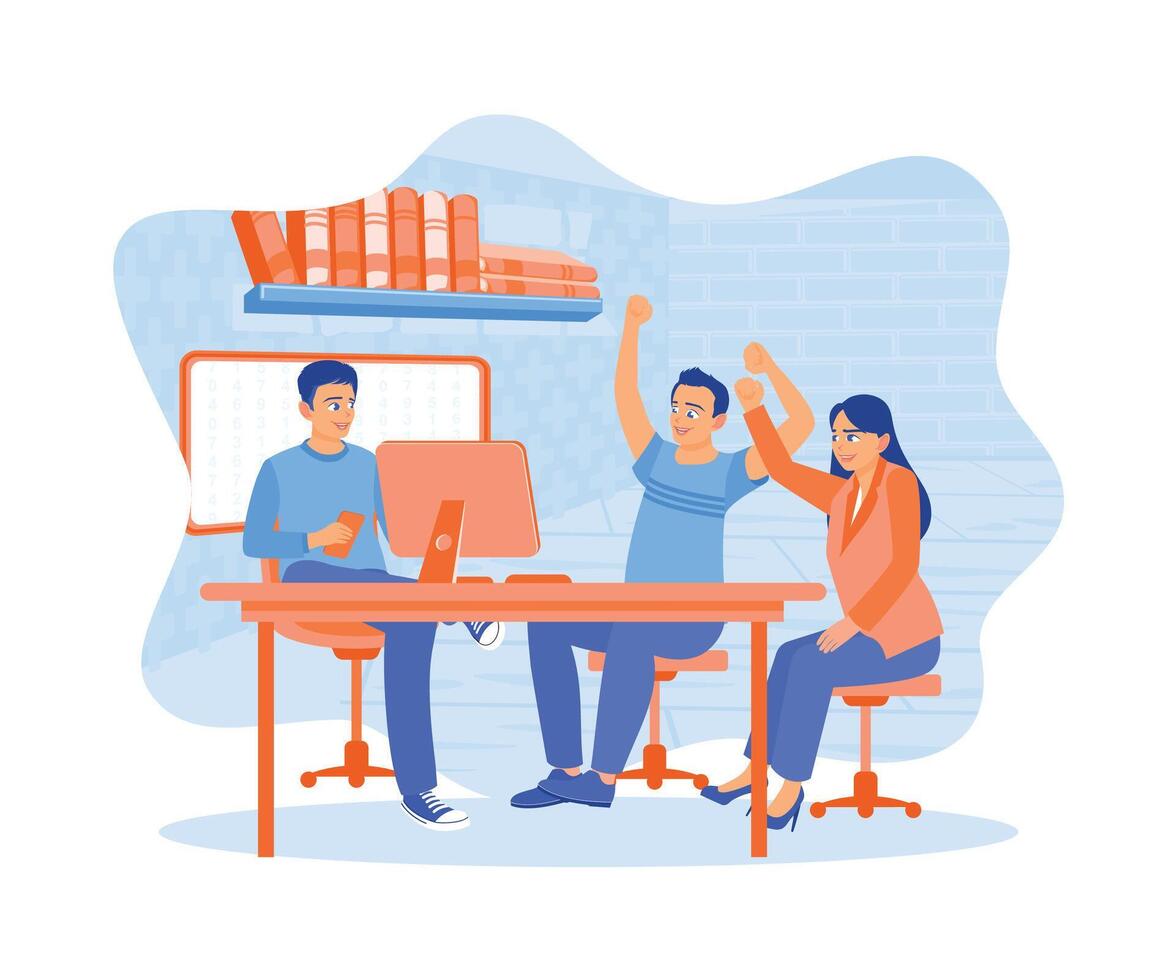This color drawing depicts three students, possibly Indian, sitting at an orange table by a large Apple LCD monitor, immersed in a celebratory moment. The background features a blue brick wall with a darker blue shelf on it, filled with thick orange and pink books. Below the shelf, there's what appears to be a whiteboard with an orange border. The room carries a generally blue tone, including a powdery blue, oval-shaped floor area. 

All three individuals are seated on small pink and orange stools, and they all wear blue pants. The woman, positioned on the right, sports an orange jacket paired with high heels and has one arm triumphantly raised in the air. The man on the left holds an iPhone in his left hand while watching his peers. The middle man, identifiable by the stripes on his shirt, has both fists pumped in the air, reflecting their collective excitement, presumably at something displayed on the monitor. The scene exudes a sense of teamwork and success, accentuated by the vibrant orange and blue color scheme.